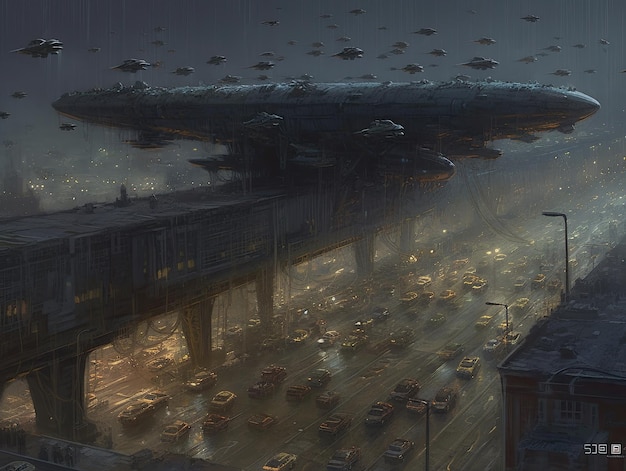In this highly detailed, computer-generated image, a bustling, futuristic cityscape is meticulously illustrated, viewed from an elevated perspective looking down on a congested 10-lane highway. Numerous sleek, futuristic vehicles fill the highway, navigating through the thick traffic. Above the highway, an elevated train track is supported by solid pillars, creating a boxed-in appearance. Perched precariously on this structure is a large, looming spaceship, giving the impression of an ominous presence over the chaotic scene below. Additionally, smaller spacecraft hover in the foggy, rain-soaked night sky, contributing to the city's dense, vertical layering. The image captures the eerie glow of vehicle lights and the muted illumination from the cityscape, painting a vivid picture of a dystopian, rain-drenched metropolis.